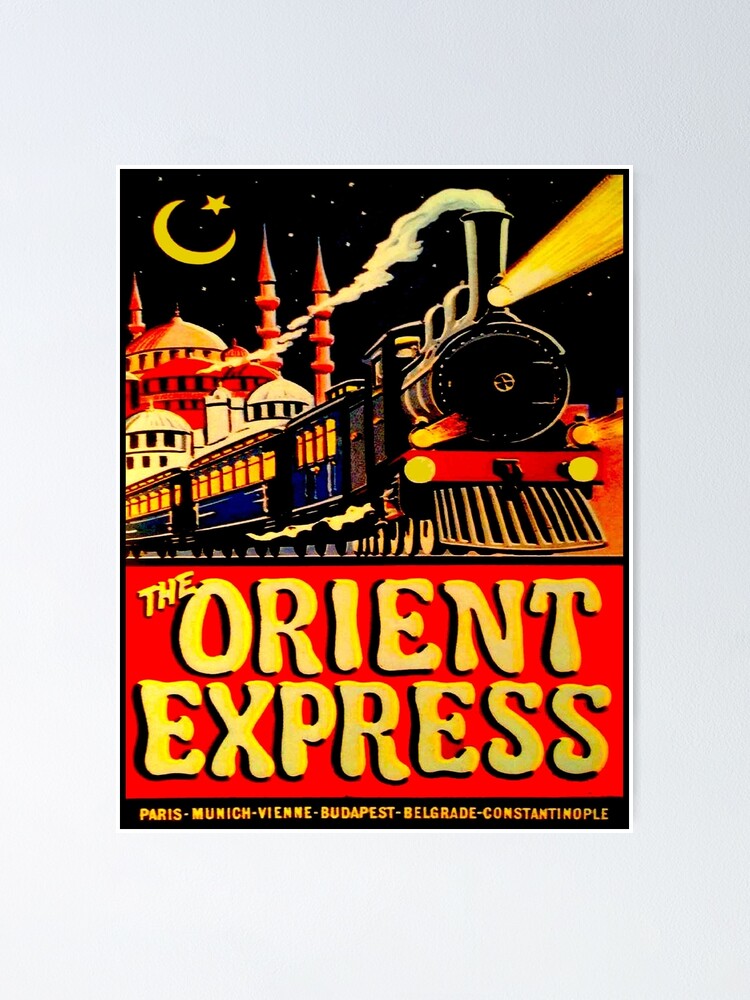The image is a vintage-style poster that likely serves as a book, movie, or magazine cover. It has a completely white background framing a square central image. The artwork itself features a black night sky speckled with white stars, a prominent crescent moon with a yellow star nestled in the curve, and a black train with a red bumper, emitting white smoke from its smokestack. The train, with its illuminated passenger cars showing blue bottoms and glowing yellow windows, is placed centrally on train tracks. To the left, there's a depiction of buildings with a castle-like structure. 

The poster's top half is predominantly black, transitioning to red on the bottom half. Beneath the train, in large yellow all-capital letters on a red background, it reads "THE ORIENT EXPRESS." Further below, a black strip contains the names "Paris, Munich, Vienna, Budapest, Belgrade, Constantinople" in smaller yellow text, separated by dots. The dominant colors throughout the poster are yellow, red, blue, black, and white, contributing to its nostalgic, old-timey aesthetic.